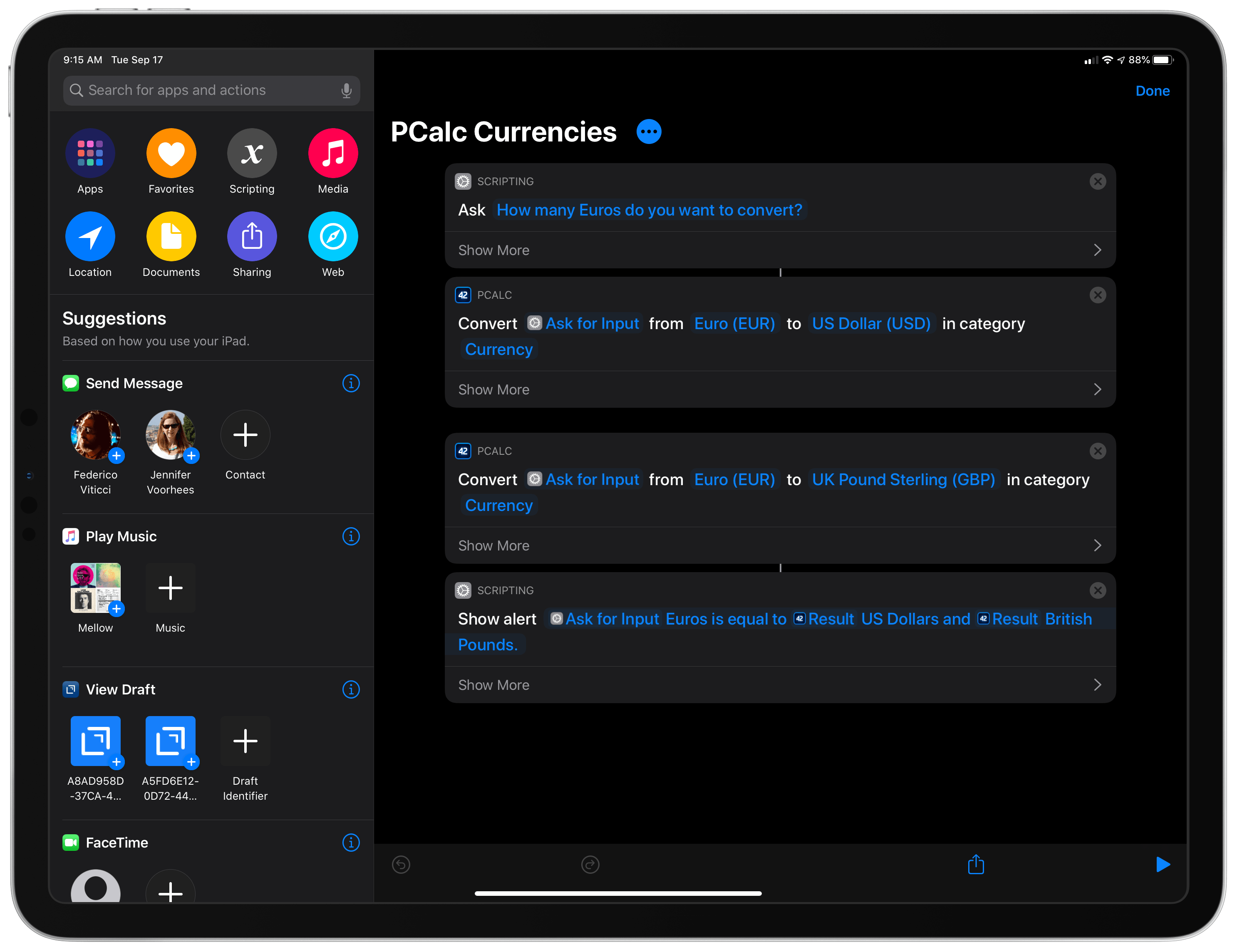A screenshot with a black background displays the time as 9:15 AM on Tuesday, September 17th. The interface shows a "Done" button on the right corner. There are eight app icons arranged in a sequence:

1. The first app icon consists of a grid of colorful squares, presumably representing various apps.
2. The second app icon is an orange circle with a white heart; the text below it is unclear.
3. The third app icon is a gray circle featuring a white 'X'.
4. The fourth app icon is a red circle with a white music note.
5. The fifth app icon is a blue circle with a white location pin or airplane symbol.
6. The sixth app icon is a yellow circle with a white numeral '7' and the label "Documents".
7. The seventh app icon is a blue circle with a white square and an arrow, labeled "Sharing".
8. The eighth app icon is a blue circle with a compass-like symbol and suggestions that say "Send the message". Additionally, two profile icons are displayed next to these suggestions.

This detailed description comprehensively covers the visible elements and layout of the screenshot.